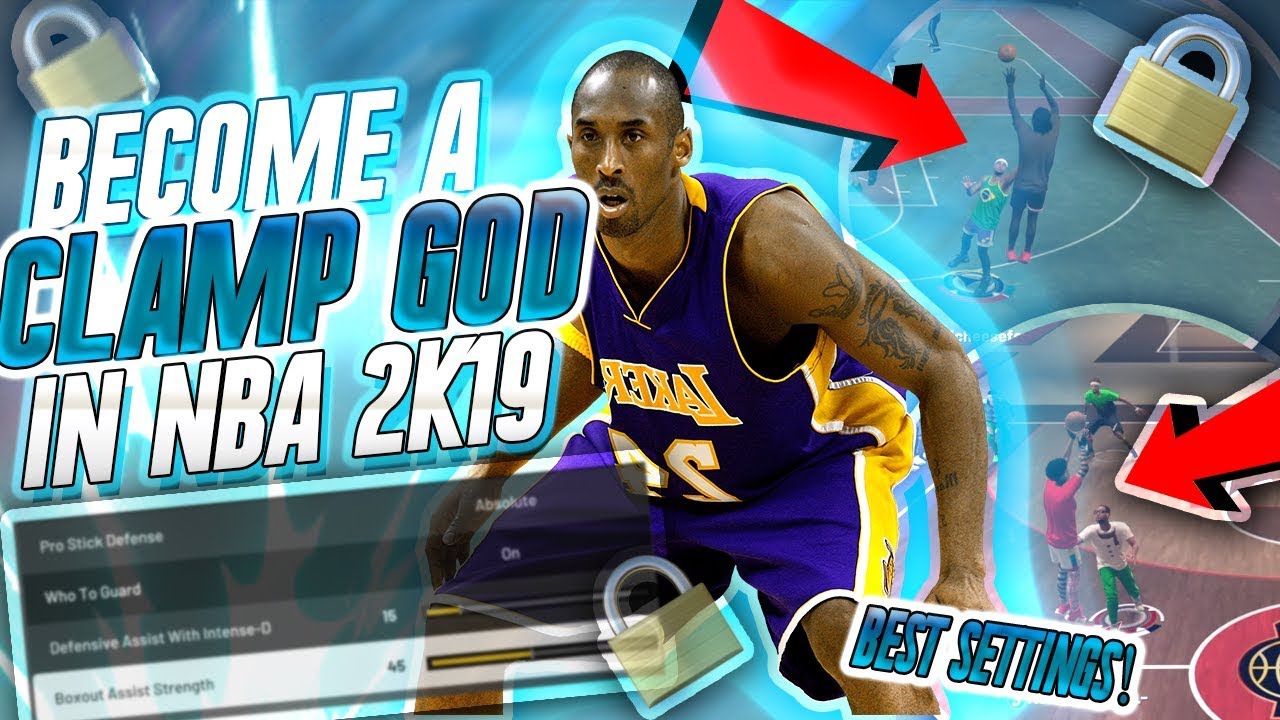This promotional image, presumably designed for a YouTube video thumbnail, centers around an African American NBA player in a Los Angeles Lakers uniform, prominently featuring a tattoo on his bicep. To his left, bold text declares "Become a CLAMP GOD in NBA 2K19," with "Become a" and "in NBA 2K19" rendered in white, while "CLAMP GOD" stands out in blue. Below this headline, an overlay of in-game settings is displayed, listing options such as Pro Stick Defense, Who to Guard, Defensive Assist with Intense D, and Box Out Assist Strength, intended for customized player settings within the game NBA 2K19.

The image is further augmented with a couple of red arrows pointing to the right, directing attention towards game footage beside the Lakers player. Scattered across the screen are three gold padlock icons, each rendered in various illustration styles, reinforcing the theme of strong defensive gameplay. In the lower right-hand corner, partially overlaying the Lakers player's leg and hand, the words "Best Settings" are prominently displayed. The image combines various visual elements to create a dynamic and engaging thumbnail, ideally suited for attracting viewers interested in NBA 2K19 gameplay tips and settings.